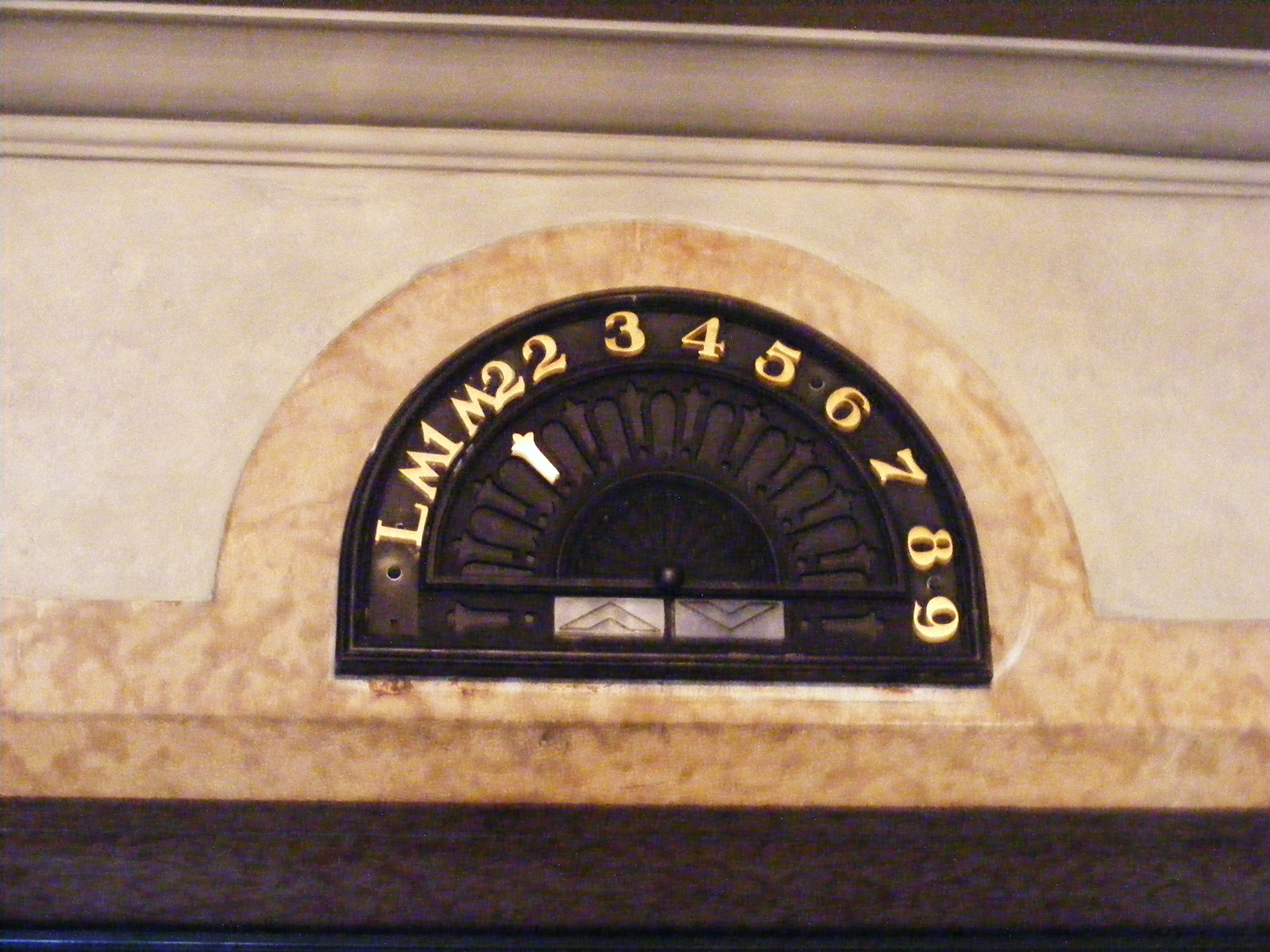The image depicts an elevator indicator panel positioned directly above an elevator door. The panel is set against a pristine white wall, framed by an elegant border made of beige stone or marble. The indicator itself is in the shape of an arched half-circle and is made of polished metal, enhancing its sophisticated appearance. It features a series of numbers and letters that trace the edge of the half-circle, starting with 'L' followed by 'M1', 'M2', '2', '3', '4', '5', '6', '7', '8', and ending with '9'. Currently, the arrow on the indicator is pointing to 'M2', signifying the elevator's position. Below the pointed arrow, there are two directional arrows, one indicating upward movement and the other indicating downward movement. At the bottom part of the image, a darker frame outlines the top of the elevator doorway, providing a visually distinct contrast to the light-colored surroundings.